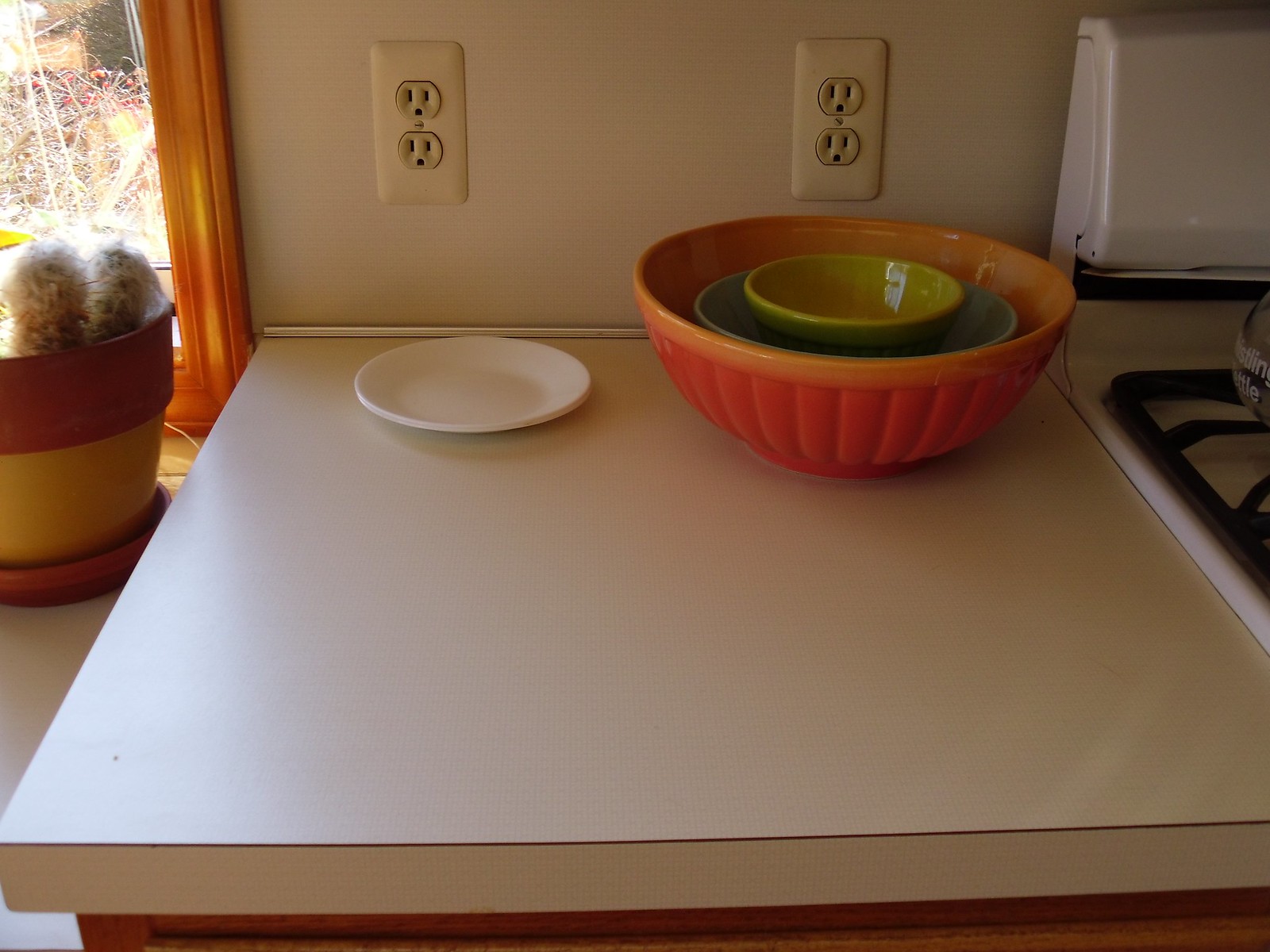In the image, there is an aged white stove with grill covers for the burners, partially visible on the right side. Adjacent to the stove on the left is a kitchen counter made of a Formica-type laminate. On the counter sits a striking orange mixing bowl, adorned with lighter orange edges and textured with puffy vertical sections creating a peaks and valleys design. Nested inside this bowl is a medium-sized green bowl with a lighter green interior and a darker green exterior. Within this is a smaller, taller green bowl featuring a similar gradient of green shades.

Beside the orange mixing bowl is a small white saucer. Further to the left, there is a lower section of the counter which holds a terracotta and yellow pot with a matching saucer. Inside the pot are two mysterious puffy white objects. A window behind the counter reveals a view of some brush outside, adding a touch of nature to the scene.